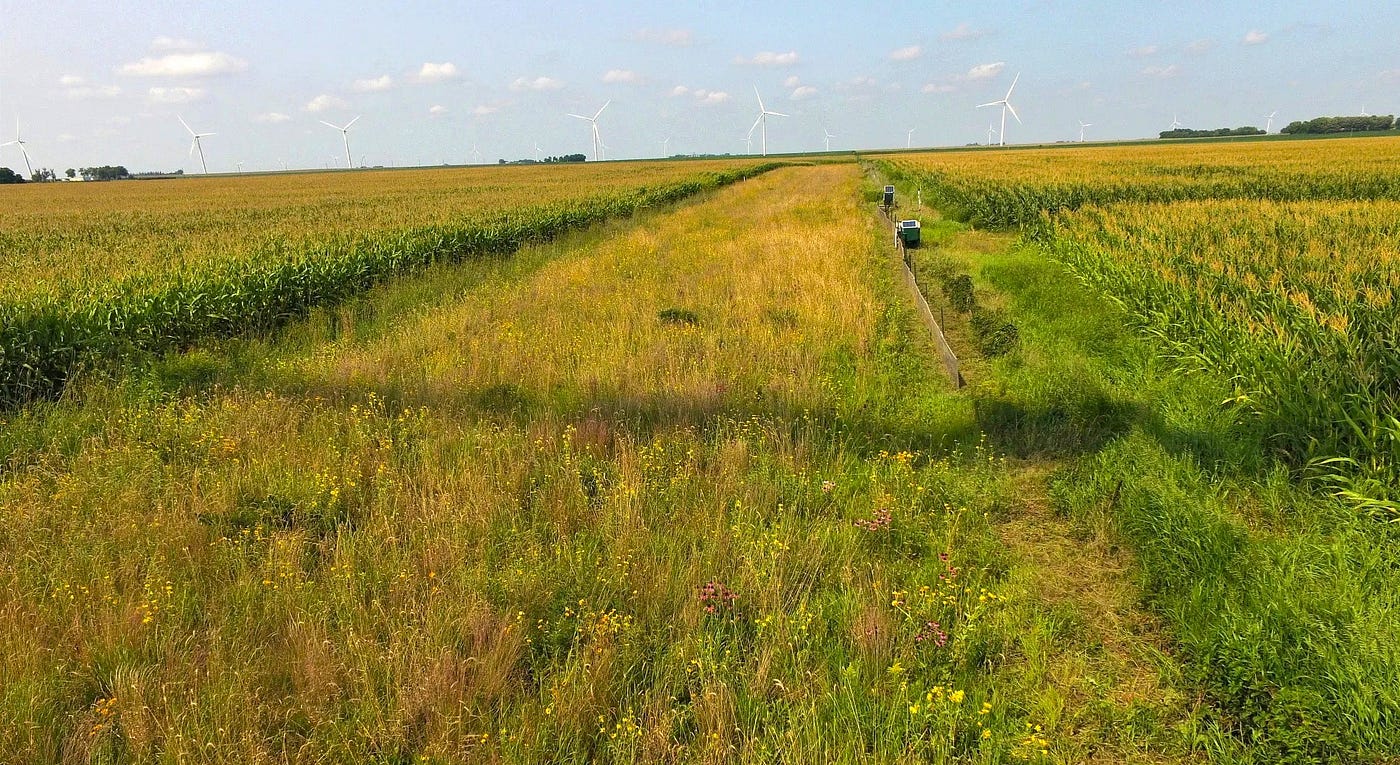This high-angle shot, possibly taken from a drone, captures an expansive field on a large farm. The photograph reveals three distinct sections: a thriving corn section on the left, a blank middle section filled with tall grasses and some weeds—possibly used for irrigation—and another corn section on the right. Both corn sections extend green, healthy stalks with flowers at the top, stretching out as far as the eye can see. A patch of greenish-grey grass hints at the onset of autumn. Bordering these sections is a partial fence that doesn't seem to run the full length of the field. Scattered around are a few large blue metal buckets for field work, and a vehicle—perhaps a truck or car—parked in the distance. Over the horizon, at least five to six tall white windmills from a wind farm punctuate the blue sky, filled with scattered clouds. The windmills with smaller ones behind indicate a larger wind energy operation adjoining the farmland. In the backdrop, faint outlines of farm structures are also visible, completing the picturesque rural landscape.